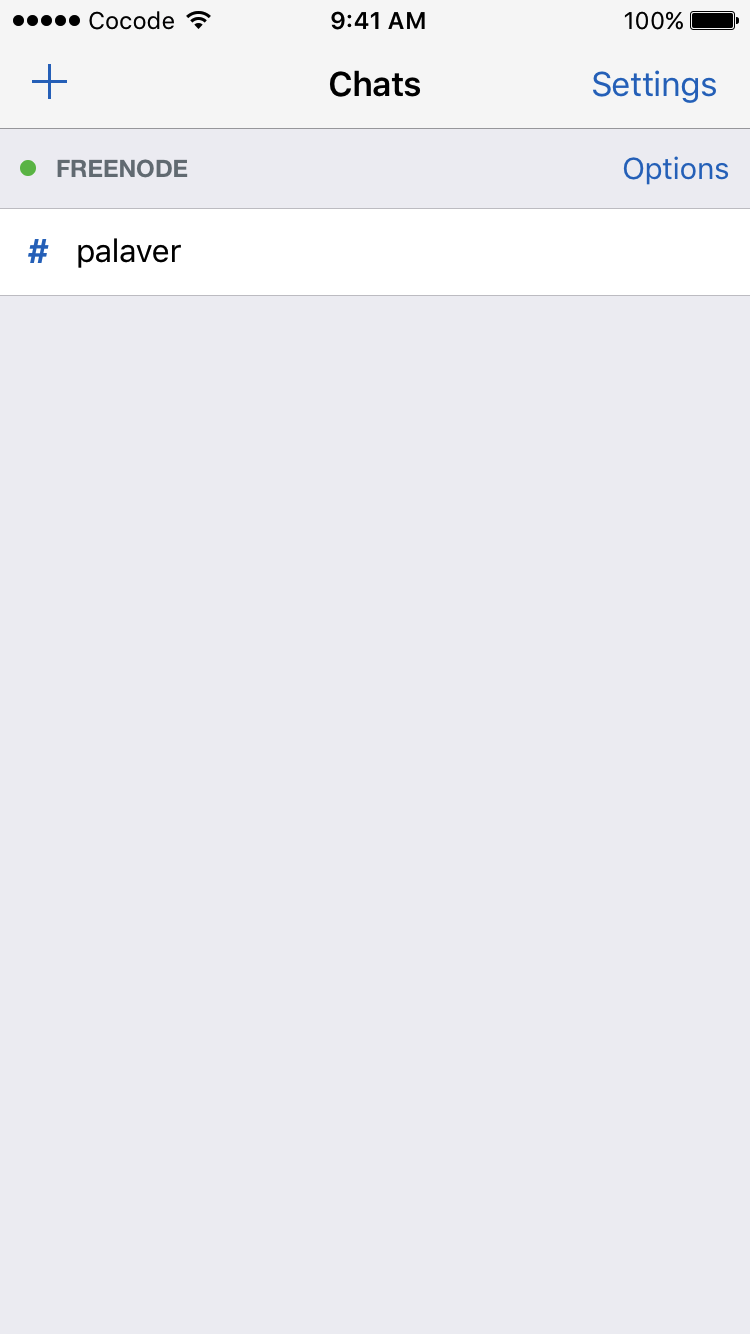The image appears to be a screenshot from a cell phone. At the top, there's a pale bluish-gray border. On the top left corner, there are five black dots, followed by the text "Co-code" and an inverted triangle icon indicating Wi-Fi. In the center, the time is displayed as "9:41 AM," and on the top right, the battery is fully charged at "100%." 

To the left of the screen, within the same section, a blue plus sign is visible. Moving to the middle portion, the word "Chats" appears in black text, and to the far right, the word "Settings" is written in blue letters. 

Below this section, there is a slightly darker grayish-blue area featuring a green dot on the left side, followed by the text "Free Note" in white. To the right of this, the word "Options" is displayed in blue letters. 

Further down, in a white section, a blue hashtag is visible on the left, followed by the word "Palaver" (spelled P-A-L-A-V-E-R). 

The bottom section of the screenshot fades from a bluish-gray at the top to a lighter color towards the bottom.